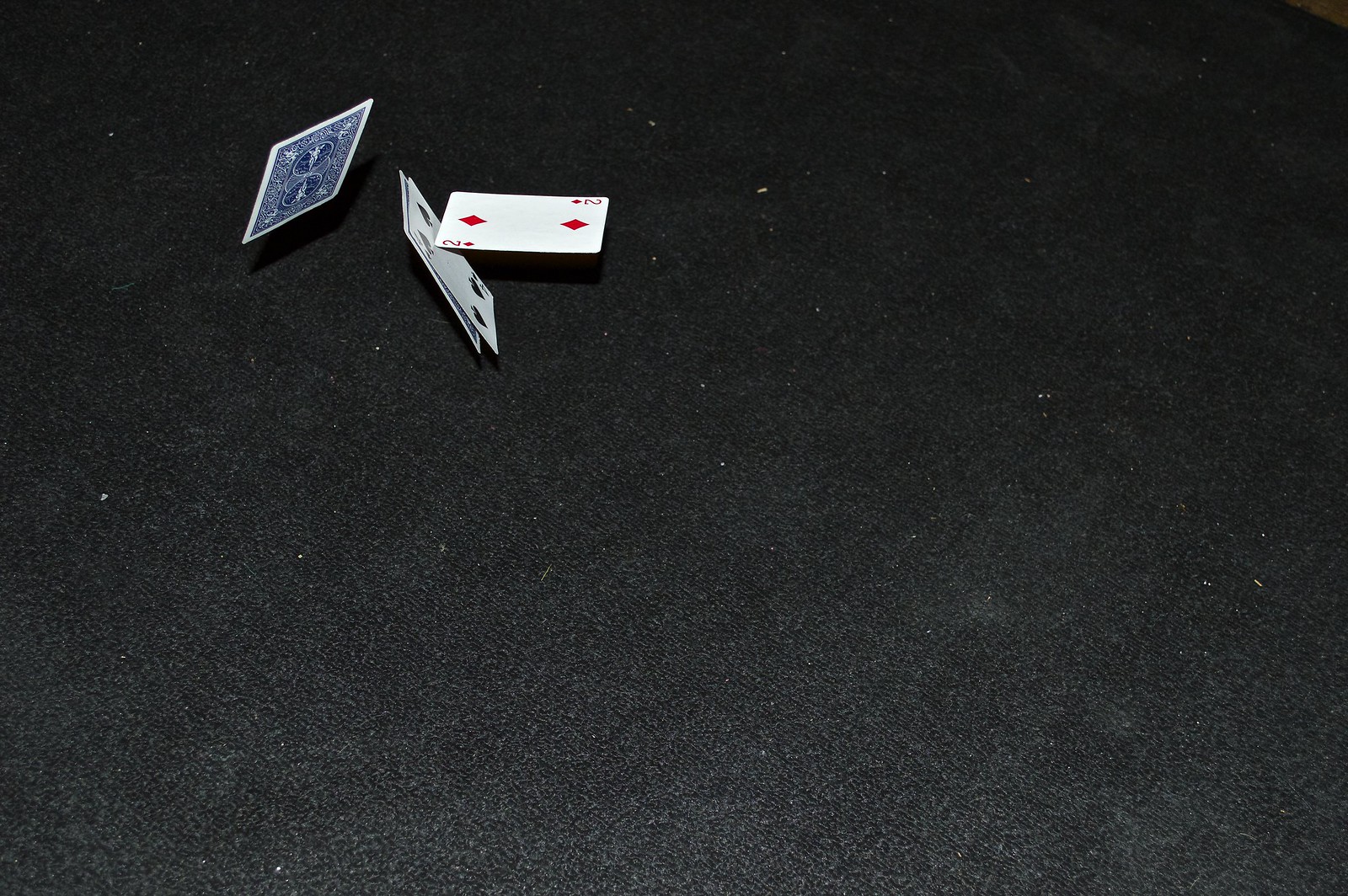The image captures four playing cards displayed against a black background, possibly a cloth, marred by a few specks of white lint. One card, predominantly blue and white, is flipped upside down and appears to be suspended in mid-air. Another card, also seemingly floating, displays the face value of 2 with red diamond symbols, positioned in front of two other cards that are angled backward. These two cards prominently feature four black spade symbols. The arrangement slants slightly to the left, with two cards appearing elevated, the blue and white card positioned higher than the others. The overall setup suggests a high-stakes, dynamic moment, as if the cards were caught in the midst of being dealt or thrown.